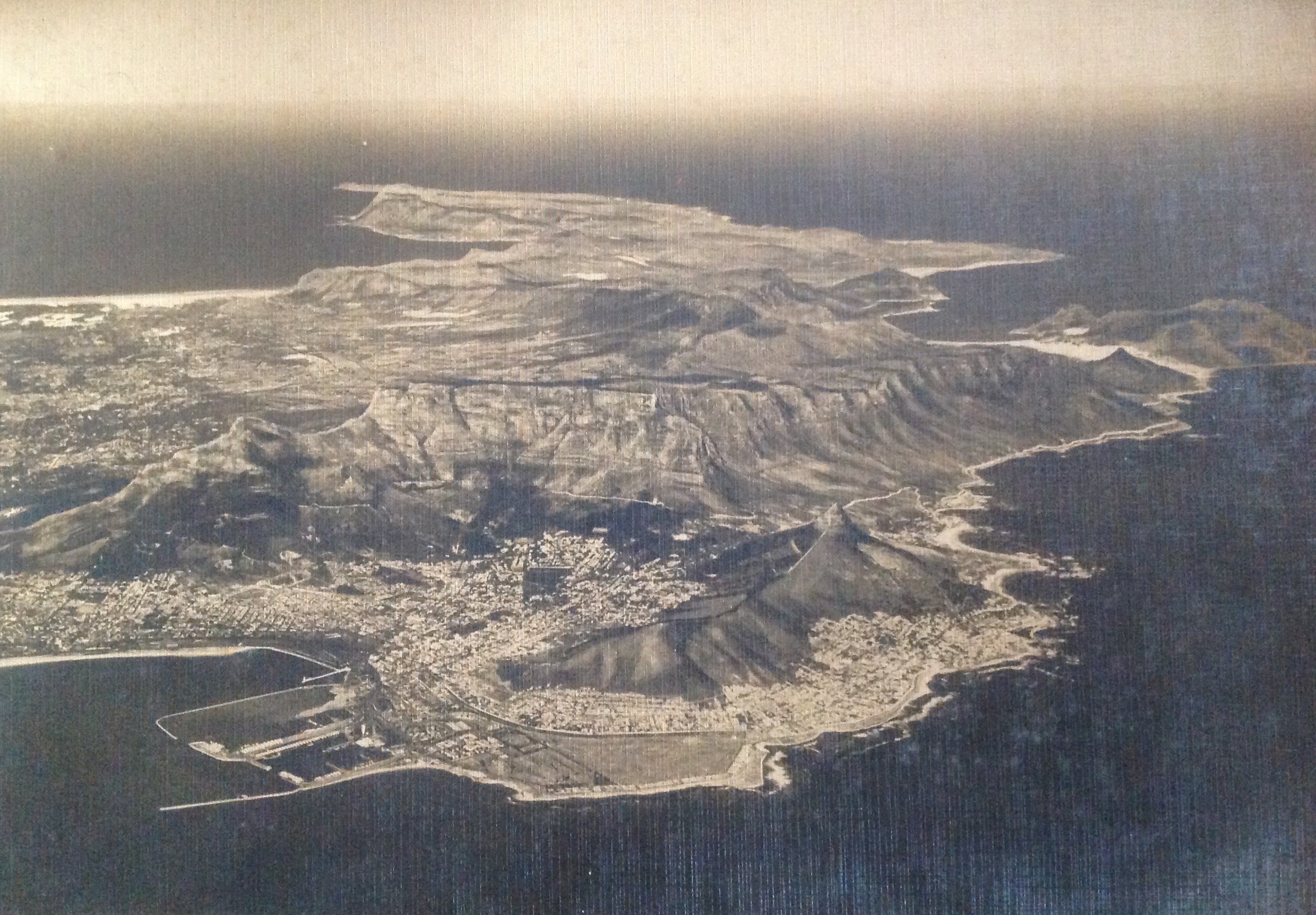This is a vintage, grainy, black-and-white aerial photograph of an inhabited island, reminiscent of the World War II era. The resolution is low, making finer details hard to discern, but several key features are distinguishable. The island is surrounded by dark, almost black water which forms a stark contrast against the gray and white tones of the landmass. A prominent mountain range occupies the center of the island, with what appear to be man-made structures at its base, indicating human habitation. Along one side of the island, there are docks and piers, suggesting the presence of a little harbor or shipyard. Though the details are small and indistinct, the coastline shows signs of a possible town or city, highlighted by white dots that could represent lights or buildings. The overall composition blends into a dark, murky sky, seamlessly merging with the ocean, adding to the photograph's aged and historical appearance.